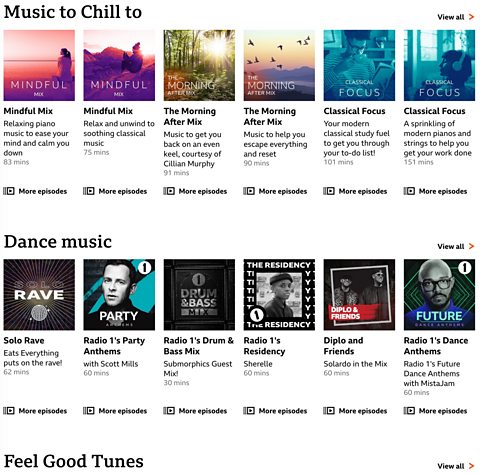A serene early morning sky, painted in soft pink hues, forms a tranquil backdrop for six neatly arranged squares. Each square represents a distinct playlist, symbolizing various moods and times of the day. A translucent purple bottle sits thoughtfully among the squares, epitomizing relaxation and mindfulness. This curated experience, featuring relaxing piano melodies, aims to soothe your mind and calm your spirit.

Named "Mindful Mix," the selected playlists range from tranquil classical music for a focused study session to uplifting modern pianos and strings to inspire productivity. Sprinkled throughout are dynamic genres such as radio anthems, drum and bass mixes, dance tracks, and DJ residencies, catering to a wide spectrum of musical tastes. Courtesy of Celia and Murphy, this collection is a family effort to offer the perfect soundtrack for any occasion. With more episodes and even more feel-good tunes, this array of twelve playlists ensures there's music for everyone, providing an auditory journey to help you regain balance and find joy in your day.